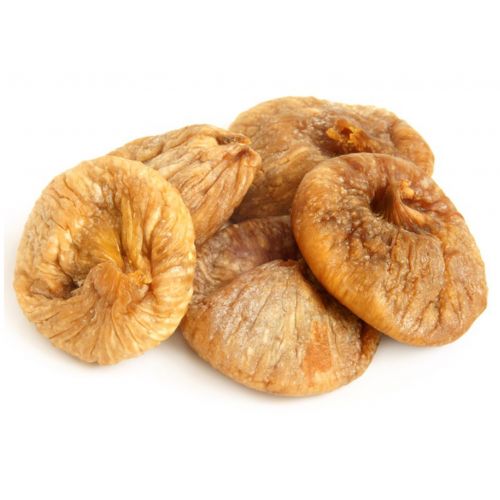In the image, there are five circular, light brown objects that appear to be figs. They are clumped together in the center-right of a completely white background, giving the impression of a simple, possibly kitchen or grocery store setting. Each fig displays a wrinkled, soft, and squishy texture, looking dried or aged. The figs are of varying shapes, with one at the bottom center being notably wider and possibly bloated. Another fig stands upright, leaning against the central one, twisted in the middle. Behind them, you can see the top of one fig resembling a wrinkled walnut. One of the figs, lying flat against the others, has a dark center where it was plucked from the stem and is particularly shriveled. The overall impression conveys a cluster of dried figs, detailed with a spectrum of brown tones from light to dark.